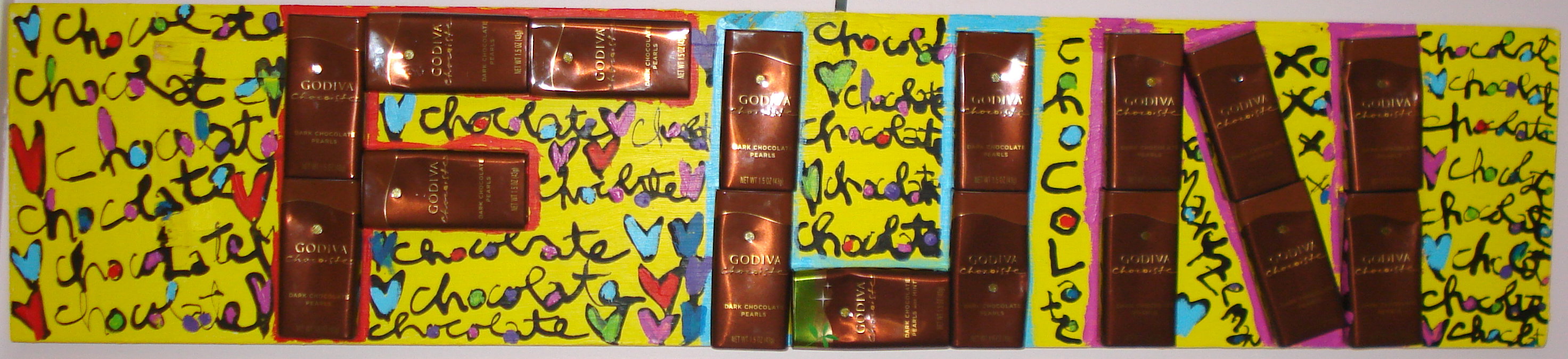In this vibrant, eye-catching photo, a creative mural captures the word "FUN" spelled out using Godiva chocolate bars. Each letter in "FUN" is meticulously formed using several brown, shiny chocolate bar wrappers, with some bars featuring hints of gold coloring and one notably opened wrapper displaying the chocolate inside. The cheerful design is set against a bright yellow backdrop, with the word "chocolate" repeatedly written in black cursive with colorful accents throughout—some letters colored in hues of pink, blue, dark blue, and light blue. Adding to the playful atmosphere, a series of hearts in various shades of red, blue, and purple are interspersed among the words "chocolate," creating a lively and whimsical artwork that merges chocolatey indulgence with artistic flair.